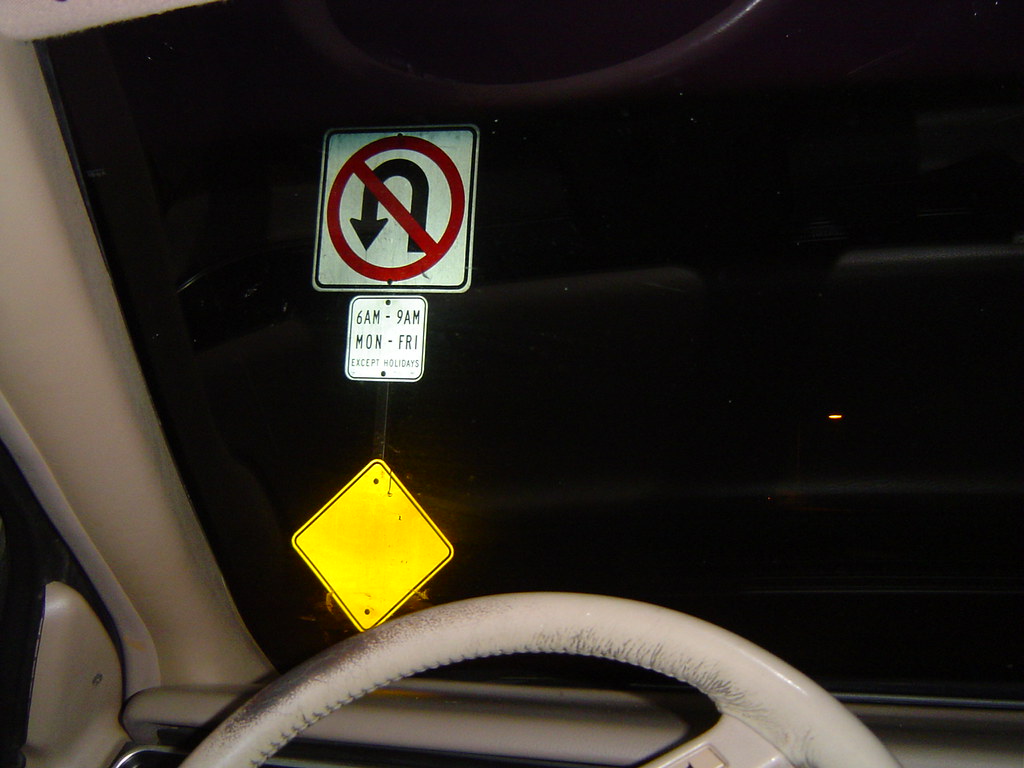The photograph, captured from the driver's seat of a vehicle, showcases the interior of the car at night. The light cream-colored steering wheel, showing noticeable wear on the top left, partially obstructs the view. The dashboard, predominantly black, is visible beneath the steering wheel, while a segment of the windshield pillar, matching the gray-beige color scheme of the interior, supports the windshield. On the bottom left corner of the image, a slight glimpse of the rearview or side mirror can be seen. Through the windshield, three illuminated road signs stand out against the dark sky. The top sign is a no U-turn sign, featuring a black arrow pointing backward with a red circle and line through it. Below it, a white square sign reads "6 a.m. to 9 a.m. Monday through Friday except holidays." At the bottom, a yellow diamond-shaped sign, devoid of any text or symbols, is prominently visible.